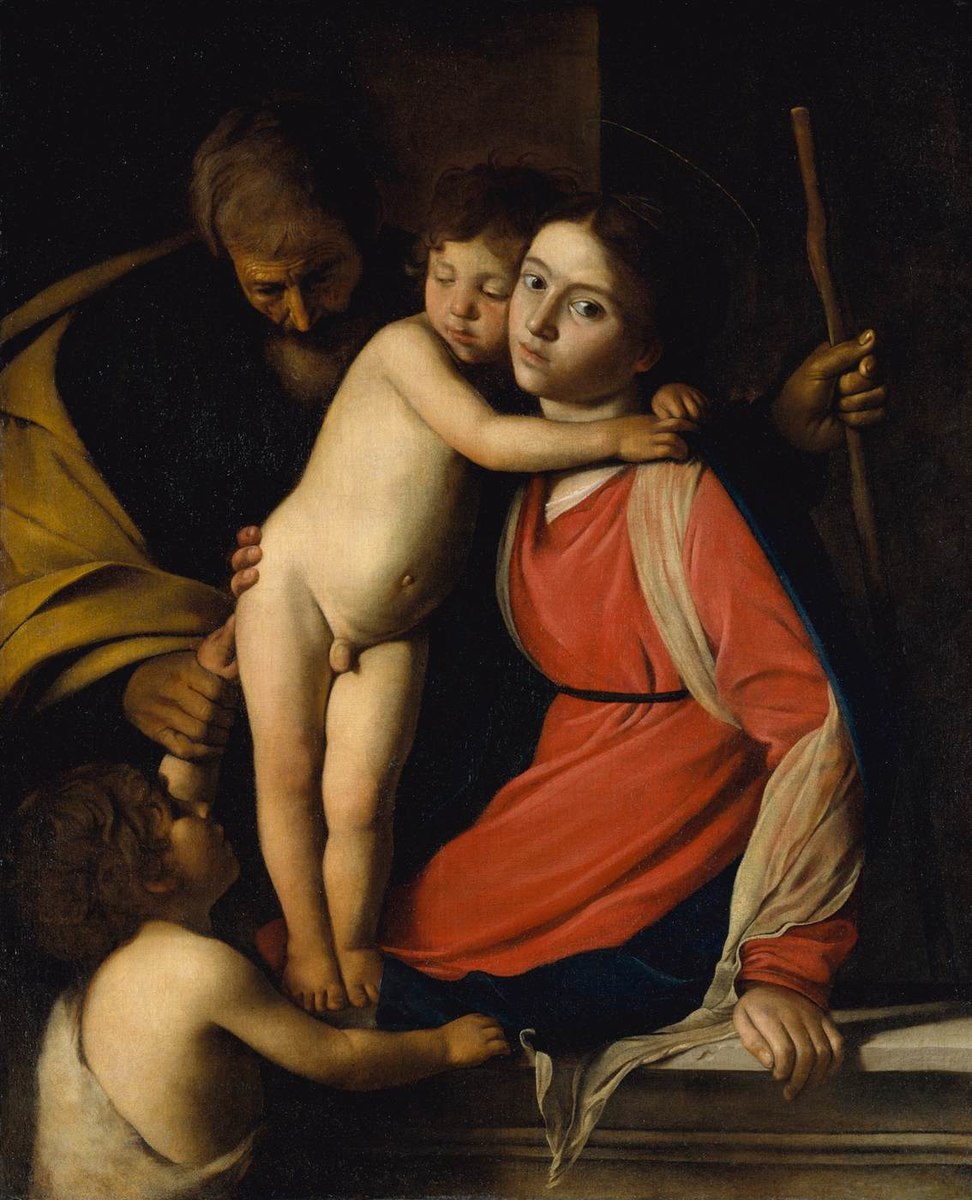This Renaissance painting features a somber woman dressed in a reddish-orange robe, accented by a beige, flowing scarf. She is seated on a marble balcony or table, gazing sideways with dark brown eyes. A nude boy, displaying red hair and male genitalia, embraces her neck while she supports him by the waist or buttocks. In the lower left corner, another child stands, looking up at this affectionate pair. In the background, mostly in shadow, stands an older, bearded man wearing a tan or olive-colored robe and holding a stick. The contrasting dark and light elements evoke the style of a Rembrandt, though it is likely not his work. The scene's central figures and composition suggest it might depict a religious subject, possibly Mother Mary with baby Jesus and Joseph.